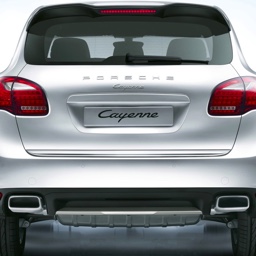This photograph captures the rear end of a silver Porsche Cayenne, prominently displaying the model name "Cayenne" in place of a license plate. The car features distinctive design elements such as black lower sections and black tires. The rear is characterized by red, oval-shaped taillights and a top-placed third brake light on the darkened rear window. Additional visible details include silver exhaust tips and a gleaming underbody, suggesting the vehicle may be on display. Although the exact text above the "Cayenne" badge is unclear, the overall setting and central placement of the vehicle enhance its luxurious presence, despite the image being truncated at the tires and lower part of the lamps.